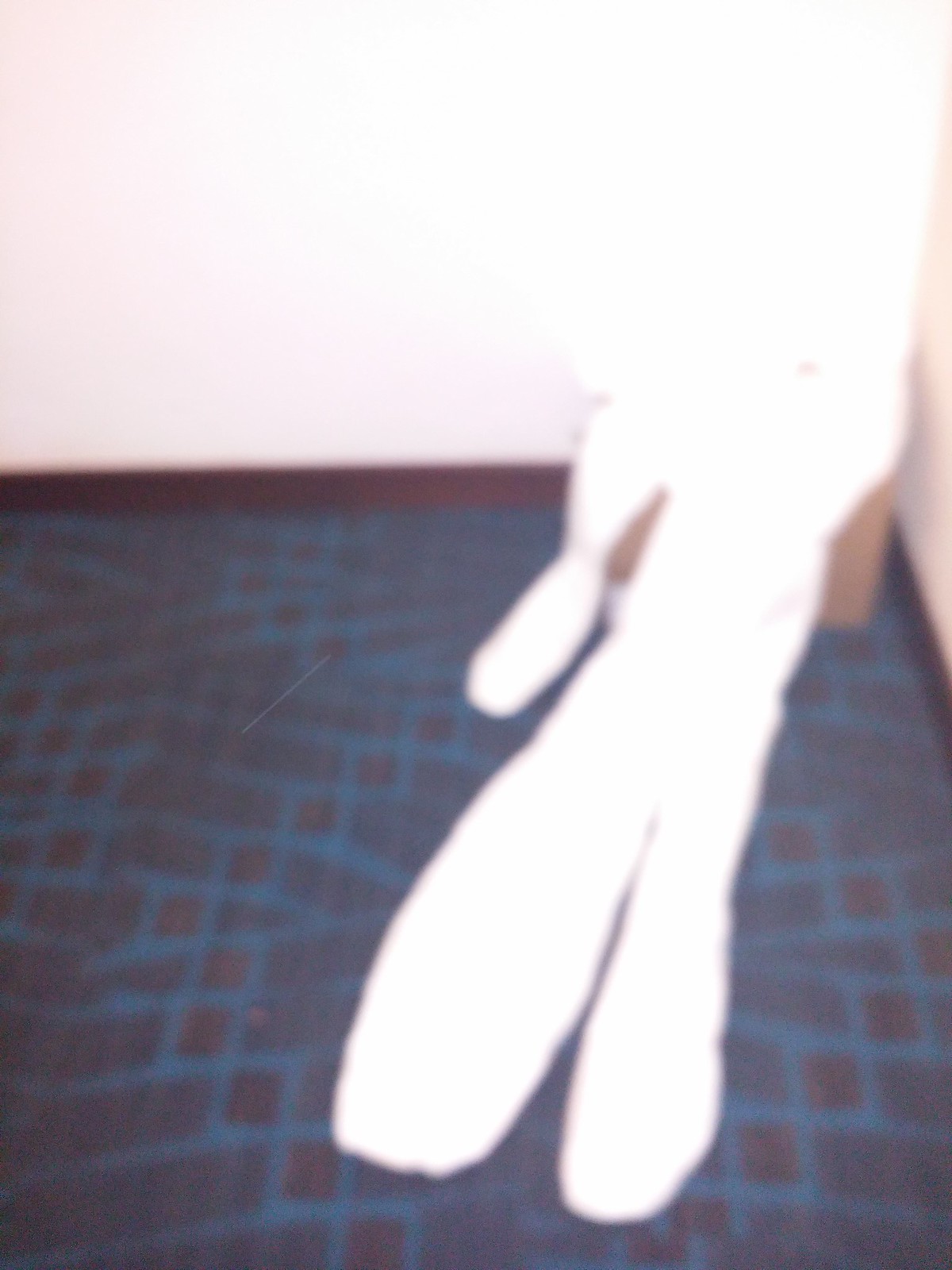This is an out-of-focus photograph taken inside a room with white, slightly beige-tinted walls and a dark mahogany or brown two-inch baseboard running around the bottom. The floor features a mix of dark red and royal blue squares in an irregular pattern, almost resembling scales or a leather-grained texture. The photograph captures the room's corner, with a brown box partially visible amidst large, white, edited scribbles that distort the scene. These scribbles are concentrated where two legs, an arm, and potentially a second person might be, hinting at an attempt to obscure a figure. The white shapes are particularly prominent, making the image appear as if someone's body, possibly with legs stretched out or crossed, has been clumsily erased or edited, resulting in a surreal and confusing composition.